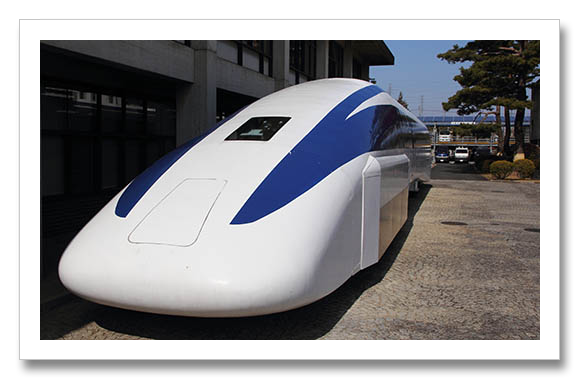This image depicts a sleek, streamlined electric bus, although it carries the appearance of a bullet train or high-speed rail car, parked in an outdoor setting. The bus is notably white with wide blue stripes running along both sides. At the front center of the bus, there is a small, vertical rectangular opening, presumably for the battery, and above it, a small square window for visibility. The side of the bus features black windows extending toward the back.

The setting is daytime, and the bus is parked on a street adjacent to a gray concrete building, which has glass windows and an arm structure visible. To the right, there are a few trees, and another building can be seen behind them. On the left of the bus, a parking lot is partially visible, adding context to the urban environment.